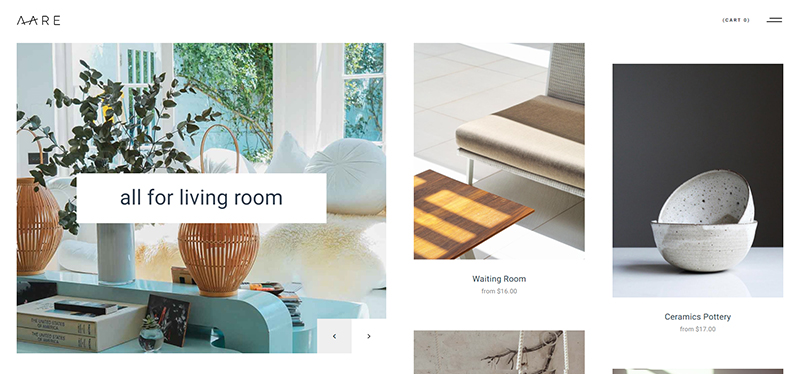This is a screenshot from a houseware store website, presumably named AARE. The screenshot features a structured layout containing four distinct photographs showcasing various products arranged across the page.

In the top left corner, the store's name, AARE, is prominently displayed. The top right corner features the label "CART 0" and is accentuated by two slim horizontal black lines along the edge.

Detailed descriptions of the photographs are as follows:
1. The photograph on the left side is square-shaped and captures a cozy room adorned with turquoise blue accents and white pillows. The room includes a collection of orange, open-woven wicker baskets and is complemented by a tall eucalyptus-like plant placed in a white vase. The large windows in the background frame a view of a clear sky and trees, adding a serene and airy touch to the scene.
2. The central photograph is in portrait orientation and depicts a bench that appears suitable for a waiting area. The bench features a brown and beige seat cushion with the back cushion rendered in an almost gray hue. The bench is supported by metal legs, and the setting rests on an off-white tiled floor. Below the bench, the text partially visible reads "Waiting room from," but the specific price is too small to discern.
3. Positioned above the photograph on the left, a white banner with the text "All for Living Room" prominently highlights the theme.
4. The photograph on the right, also in portrait orientation, contrasts with a white base and a black background, displaying two gray speckled pottery bowls. One bowl is artfully propped up inside the other, showcasing the intricate design and texture of the pottery.

This assortment of images and text combines to offer a diversified glimpse into the houseware products available at AARE.